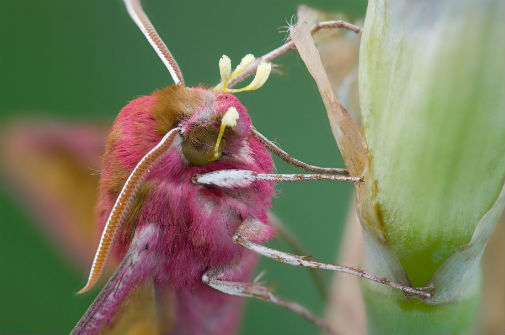This professionally shot, full-color, close-up nature photograph captures a captivating moment in a horizontally rectangular frame with no borders. The image showcases a furry insect, likely a type of moth, clinging to a green stem or bud of a flower. Set against a blurred backdrop of out-of-focus vegetation, the insect, taking up most of the center left area, is detailed with prominent antennae and is characterized by a striking blend of white, pink, and brown fur. Its body, an oval shape, features long, white legs that grip the green stem horizontally. The right side is dominated by what appears to be the insect's cocoon, colored white and green, emphasizing the emergence of this remarkable creature.